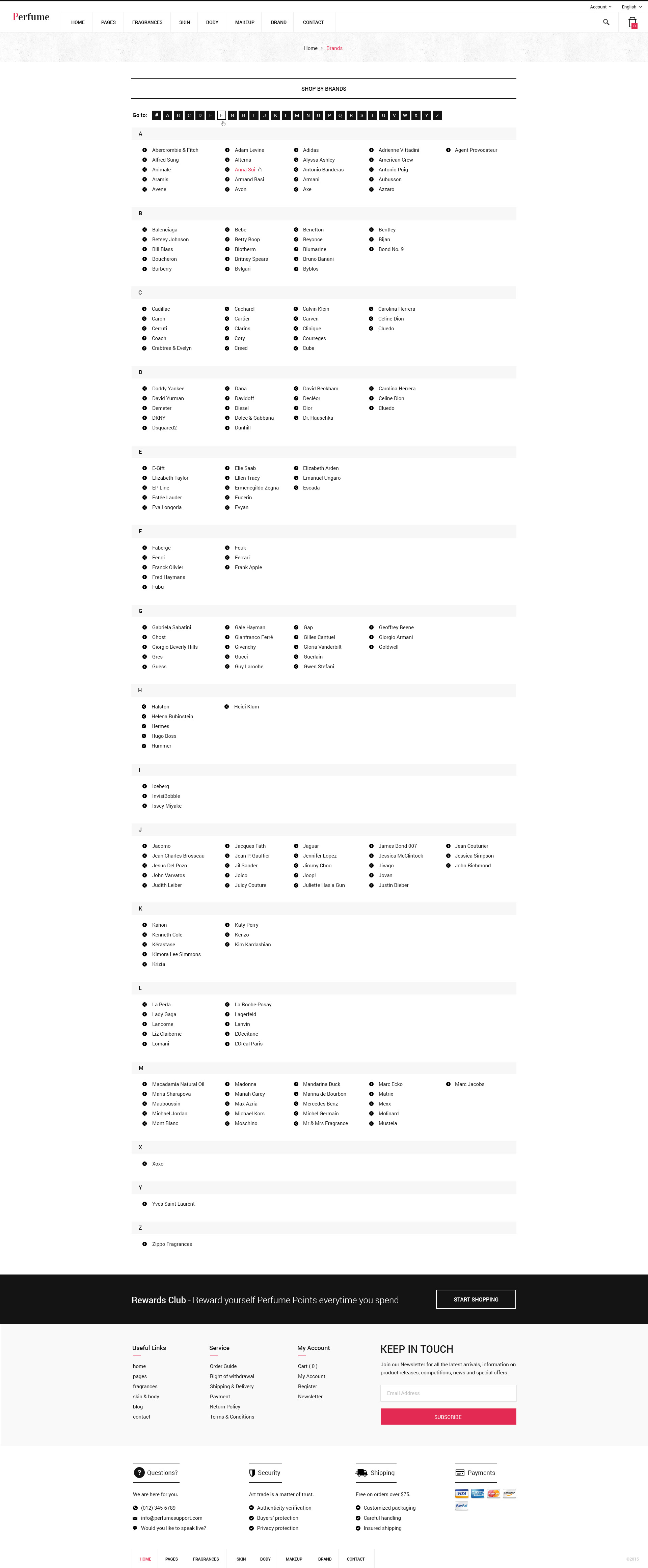The image is a screenshot of an extensive web page with a predominantly white background. The top header section, matching the background color, features a thin line at the top. The menu items, rendered in black font, are aligned horizontally across the header. Despite the small size of the image, making the text illegible, it's evident that there are seven menu items. The far-left menu item likely represents the company's name.

Below the header, the main content of the page consists of a chart-like structure, divided into four columns and four rows. These rows are separated by very light horizontal gray lines, organizing the content neatly. Although specific details of the chart are not discernible, the structured layout is clear.

Towards the bottom of the page, there is a prominent bold black horizontal line, signifying a transition to the footer section. Within the footer, on the right side, the text "Keep in touch" is visible alongside a long rectangular field for entering an email address, presumably for subscribing to a newsletter. Below this input field is a noticeable red button. In the bottom right corner of the footer, there are recognizable logos for American Express and MasterCard, indicating supported payment methods.